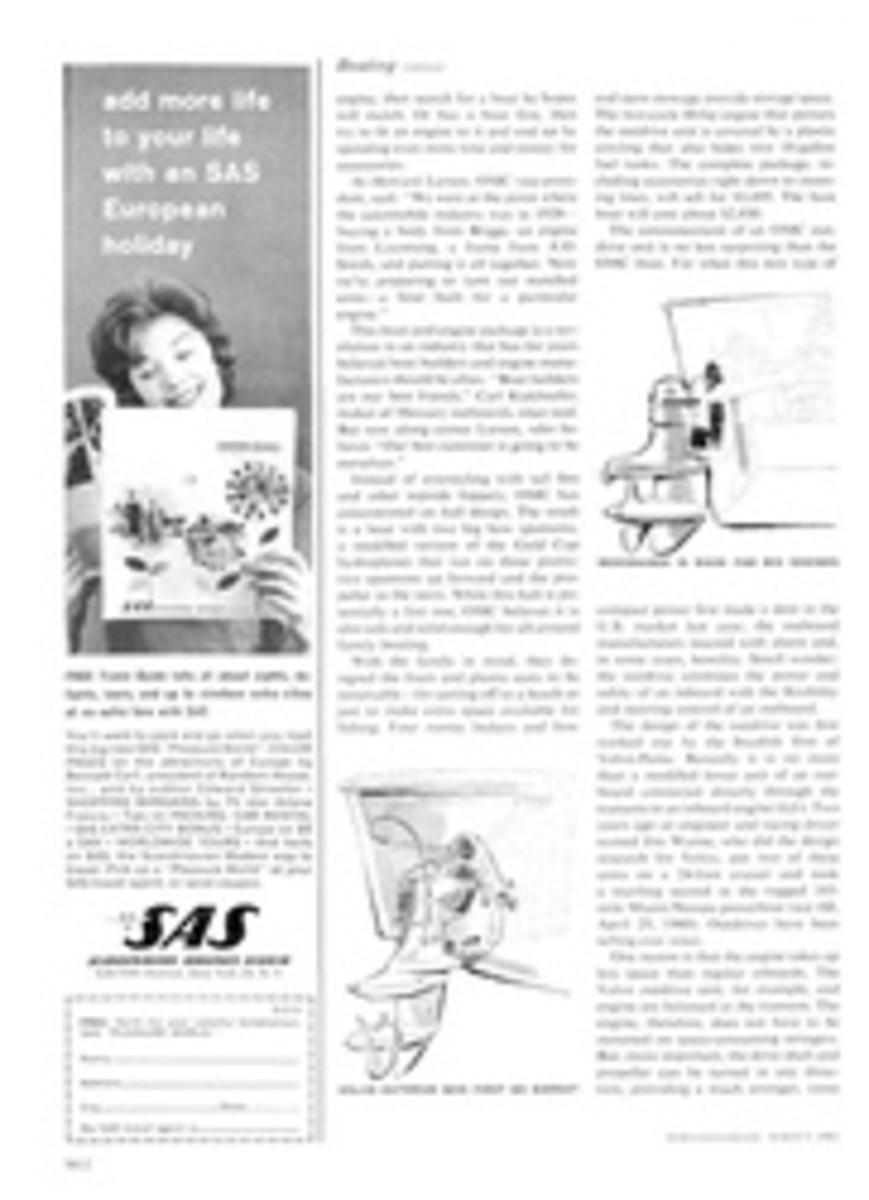This is a blurry page from a magazine, predominantly featuring text and a couple of illustrations. The main focus is a black-and-white image of a woman looking at a magazine, positioned on the left side. Above her, there's a partially legible slogan in white text that seems to read, "Add more life to your life with an SAS European holiday," followed by the bold block letters "SAS," and a small, fillable and detachable section for sending in. Along the right side, there are two columns filled with text that are too small and out of focus to read clearly. The third column consists purely of text, interspersed with some scribbling and a small, indistinct drawing.